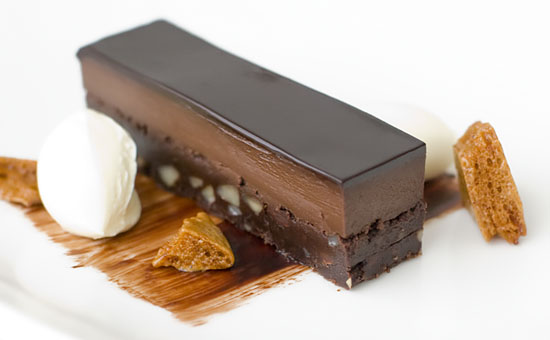This close-up photograph showcases an exquisite chocolate mousse cake, elegantly presented on a white plate. The cake is composed of two distinct layers: a darker, dense fudge-like base embedded with visible nuts, likely pecans, cashews, or walnuts, and a lighter, creamy chocolate mousse layer on top. The entire dessert is finished with a glossy dark chocolate glaze that provides a shiny, almost mirror-like finish. Beneath the cake is a decorative smear of rich chocolate sauce, enhancing its visual appeal. To the left of the cake, there is a white dollop, possibly whipped cream or ice cream, contributing a contrasting texture and temperature. Scattered around the dessert are pieces of broken cookie, adding a crunchy element. The meticulous setup not only emphasizes the decadence of the chocolate dessert but also accentuates the complementary garnishes, creating a visually appealing and mouth-watering presentation.